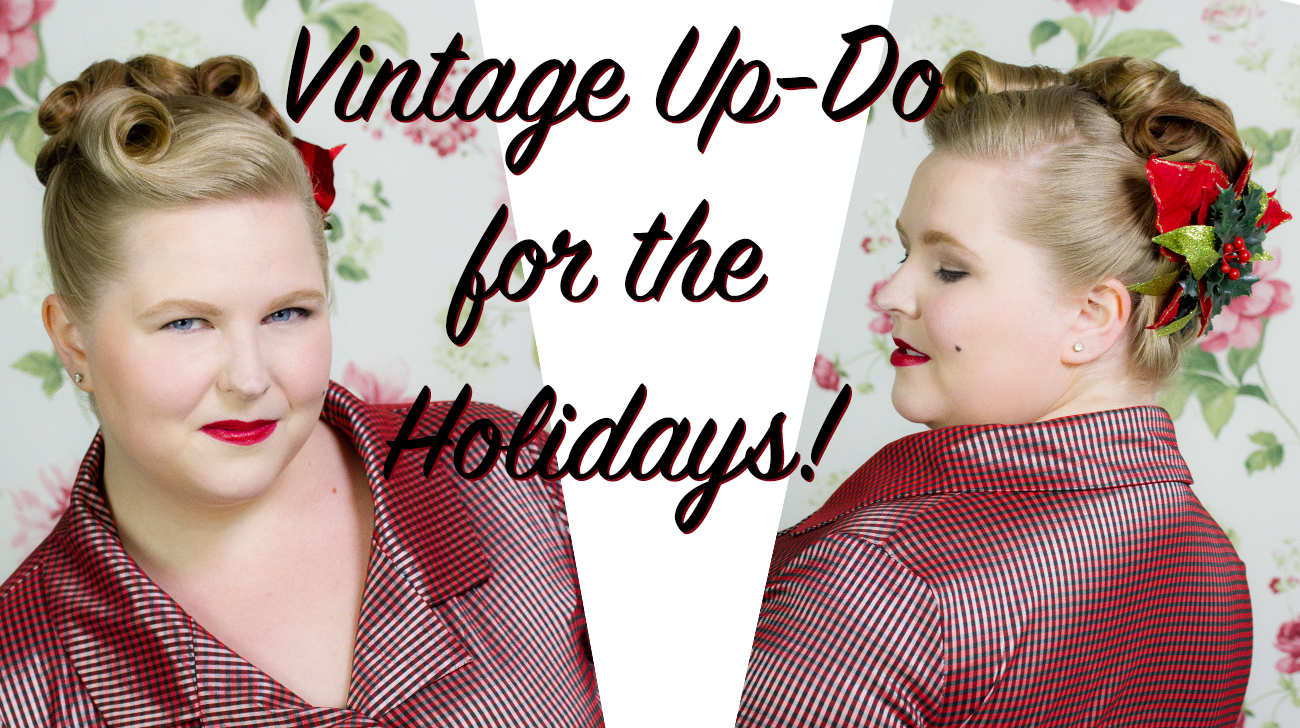The image showcases a portly woman promoting a vintage hairdo for the holidays, with two photographs of her side-by-side, divided by a white, downward-pointing triangular shape. The woman, who has blue eyes and blonde hair styled in an elegant vintage updo reminiscent of the 50s and 60s, is wearing a shiny, red, plaid shirt with black stripes. Her hairstyle features curls above her forehead and at the back, adorned with a holiday-themed poinsettia. She wears deep red lipstick, adding to the retro look. The left photograph presents a frontal view where she looks straight at the camera, standing against a white backdrop with floral print. The right photograph offers a side and rear view, emphasizing the intricate curls and the festive poinsettia in her hair. In the center, black cursive text with a red outline reads "Vintage Updo for the Holidays" across three lines, completing the vintage holiday aesthetic.